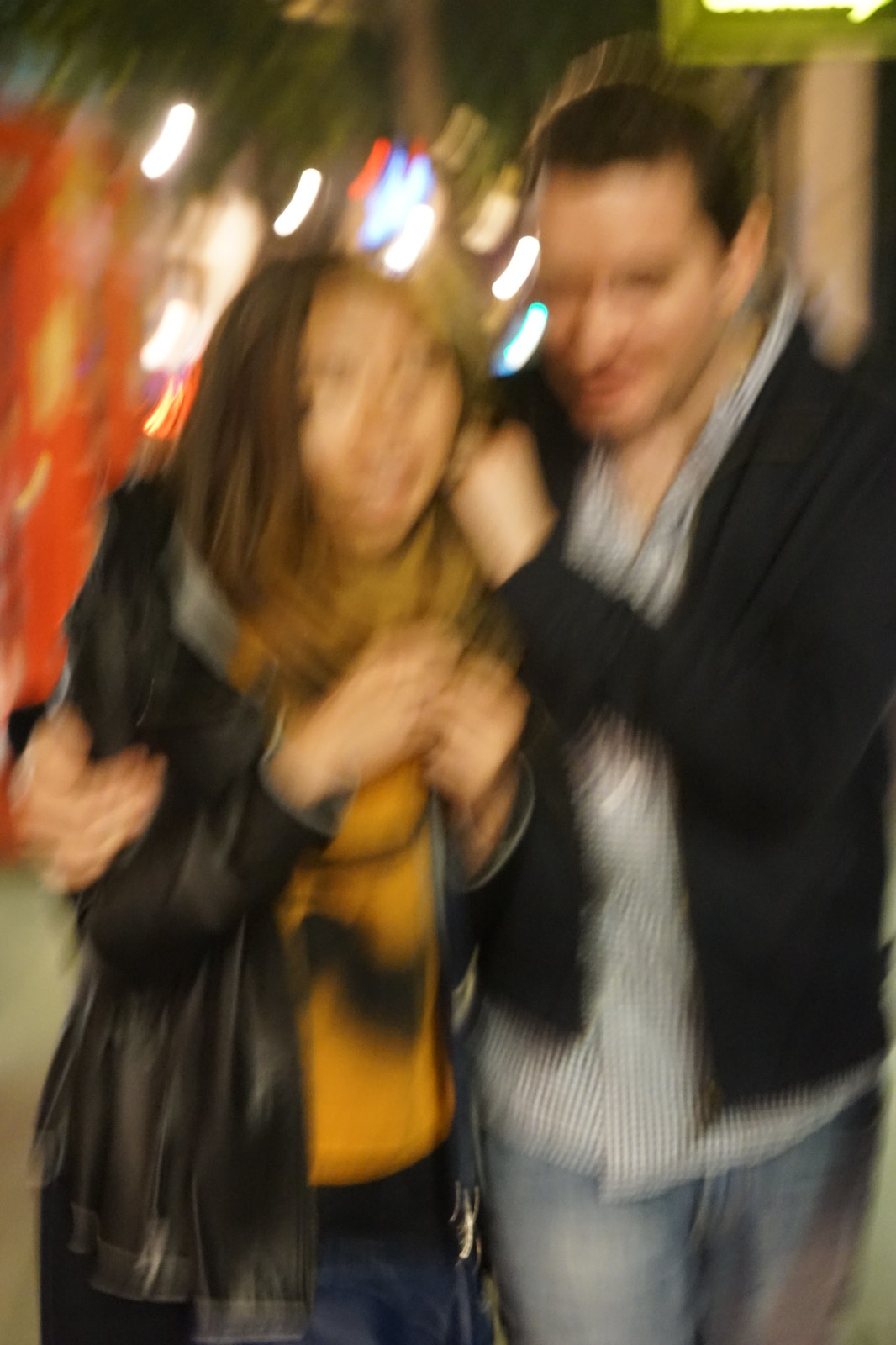A blurry image captures a man and a woman posing together on a sidewalk. The man, with short hair and a slight stubble, has a fair complexion and is wearing a white button-up shirt adorned with blue polka dots beneath an unzipped black jacket. He has a firm grip around the woman, pulling her close, which seems to make her appear somewhat uncomfortable. Her body language, with her hands tucked in, suggests a mix of surprise and discomfort. She is dressed in a black leather jacket over a gray sweater, with a visible scarf of indistinct color, possibly yellow, black, or gray, due to the blurriness. The woman, who seems to be of Asian descent, complements his attire with stylish layers that remain unzipped. In the hazy background, there appears to be a red London telephone booth, indicating a setting in a public urban space.